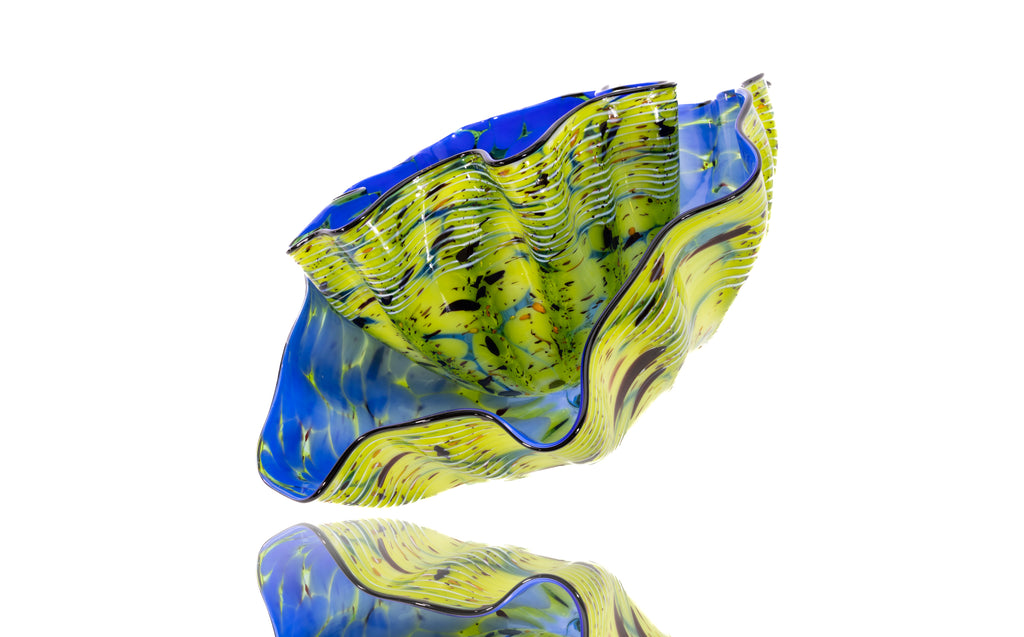The image features a set of unique, shell-like bowls with a striking, colorful design placed against a plain white background. The larger bowl exhibits a squiggly, curvy shape with high sides. Its exterior is predominantly yellow adorned with black and blue splatters, while the interior showcases a dark blue hue accentuated with wavy yellow streaks, creating a vibrant contrast. Nested within the larger bowl is a smaller bowl mirroring the same intricate pattern and dynamic squiggle along the rim. The reflection of these bowls is visible at the bottom left-hand corner of the image, enhancing the composition. The third partial bowl appears at the bottom, continuing the consistent color scheme and design, albeit partially cut off from the frame. The detailed and lively colors give the pottery an almost floating appearance, emphasizing its glass-like quality and artistic craftsmanship.